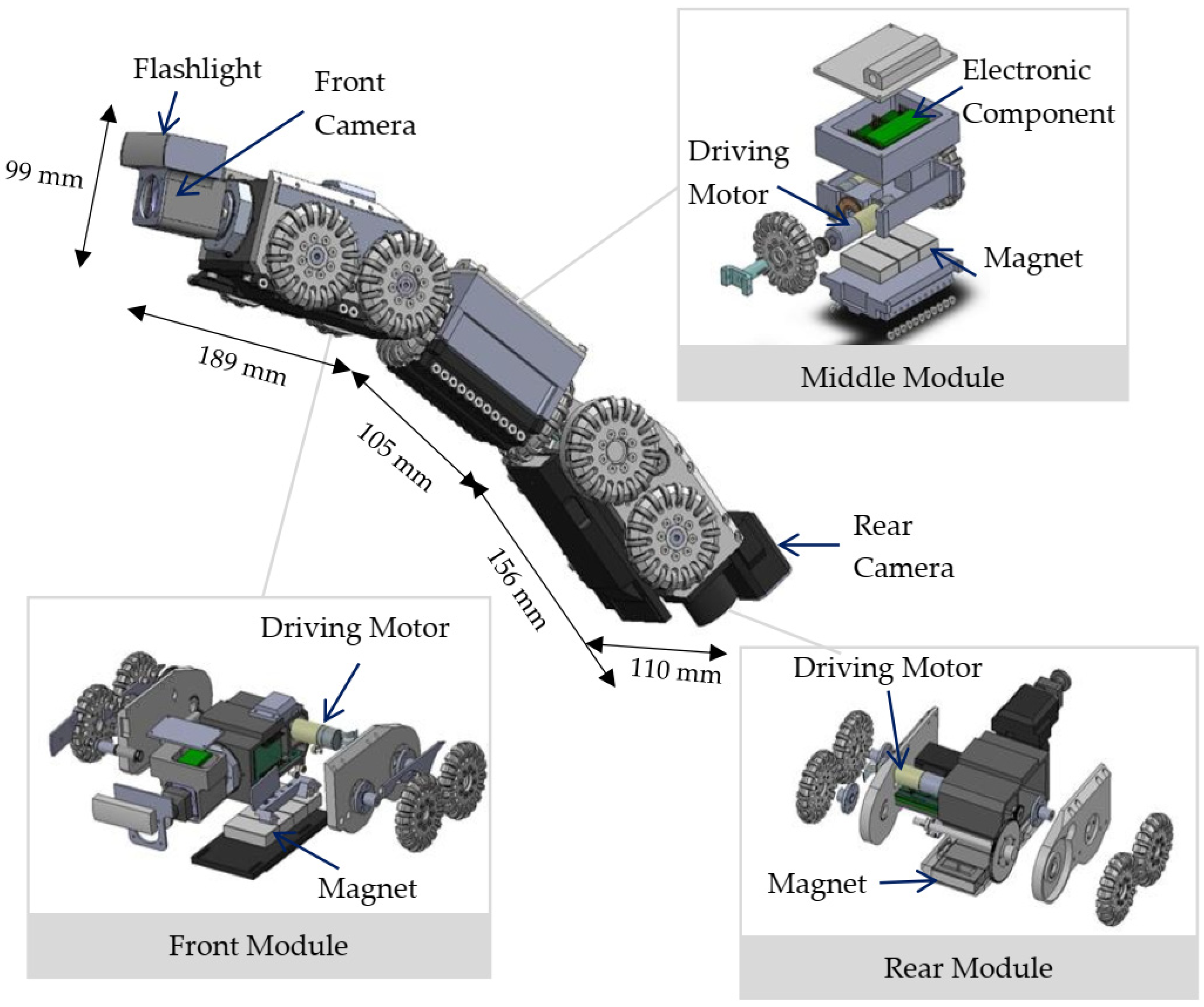This image, primarily in shades of black and gray, depicts a detailed digital illustration of various labeled components of a machine, likely used for educational purposes. The machine is comprised of several modules with individual parts clearly demarcated and labeled. 

Starting from the top right of the image, there is a section labeled "Middle Module" containing intricate electronic components including magnets and a driving motor. Adjacent to this, on the left side, there's a depiction of various camera components—front camera, rear camera, and flashlight—with their respective sizes specified as 99 mm, 180 mm, 105 mm, 156 mm, and 110 mm. 

Further, on the left side of the image, a section labeled "Front Module" illustrates parts such as a driving motor and magnets. Moving to the bottom right, another labeled section, "Rear Module," also highlights a magnet and a driving motor. 

These different modules and components are enclosed within distinct rectangular boxes, which are separated and connected with lines for clarity. The structured layout and detailed labeling facilitate a comprehensive understanding of the machine's parts and their configuration.